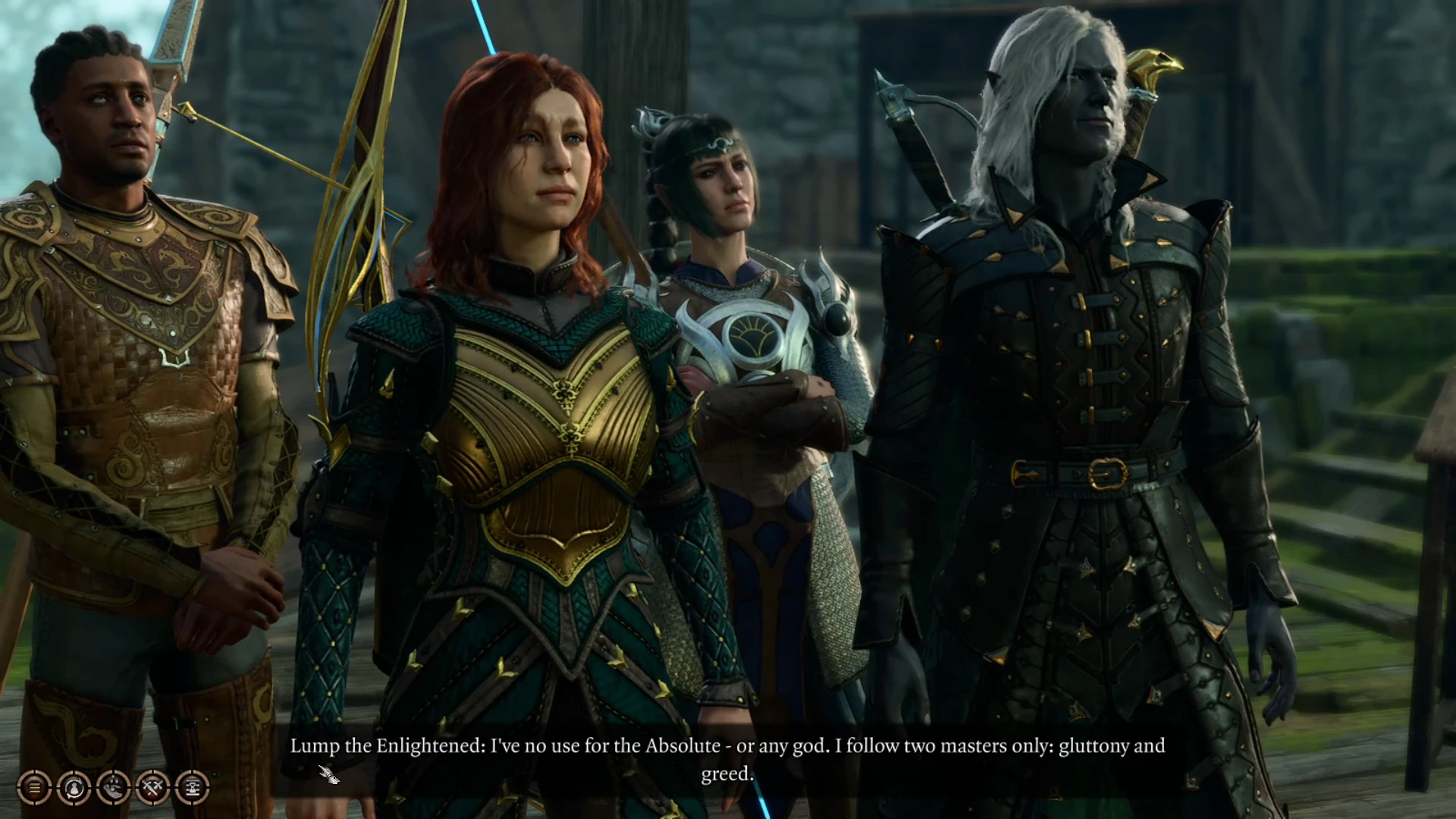The image portrays a group of four digitally contrived characters standing in what appears to be a medieval or fantasy setting with wooden stairs and possibly a castle backdrop, reminiscent of a video game or cinematic scene. Each character is adorned in distinctive armor and carries various weapons. 

To the far right stands a character with white hair, dark gray skin, and pointy ears, resembling an elf. He dons black armor and wields two swords strapped to his back, giving him a samurai-like appearance. Next to him, a female figure at the front features reddish hair, a green tunic partially covered by bronze armor, and a bow fastened to her back. 

On the far left is a man with cornrows, dressed in brown and goldish bronze armor, appearing to be African-American. Behind these characters is another woman with light skin and a ponytail, wearing face armor.

The scene includes intricate and photorealistic graphics, particularly emphasizing the character to the right. At the bottom of the image, a text box reads, "Lump the Enlightened: I have no use for the absolute or any god. I follow two masters only, gluttony and greed." This text aligns with in-game UI elements, such as character dialogue and status icons.